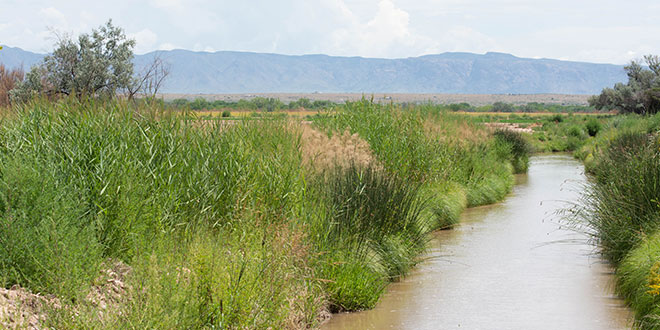This photograph captures a small, narrow, and muddy stream winding through a grassy landscape on a clear, sunny day. The stream is bordered by very tall grasses that sway gently, indicating a light breeze. The grasses vary in shades of green, with some appearing dry and tan, giving the landscape a somewhat parched look. On both sides of the stream, you can see a mix of green weeds, bushes, and a few plants. There is a noticeable strip of bare, brown dirt or sand stretching horizontally across the scene. In the far background, greenish-brown trees dot the landscape, leading up to the bluish-gray mountains that rise under a clear sky. Off to the right, there is more dense brush and an additional tree stands prominently in the top left corner, completing this serene yet slightly barren countryside vista.